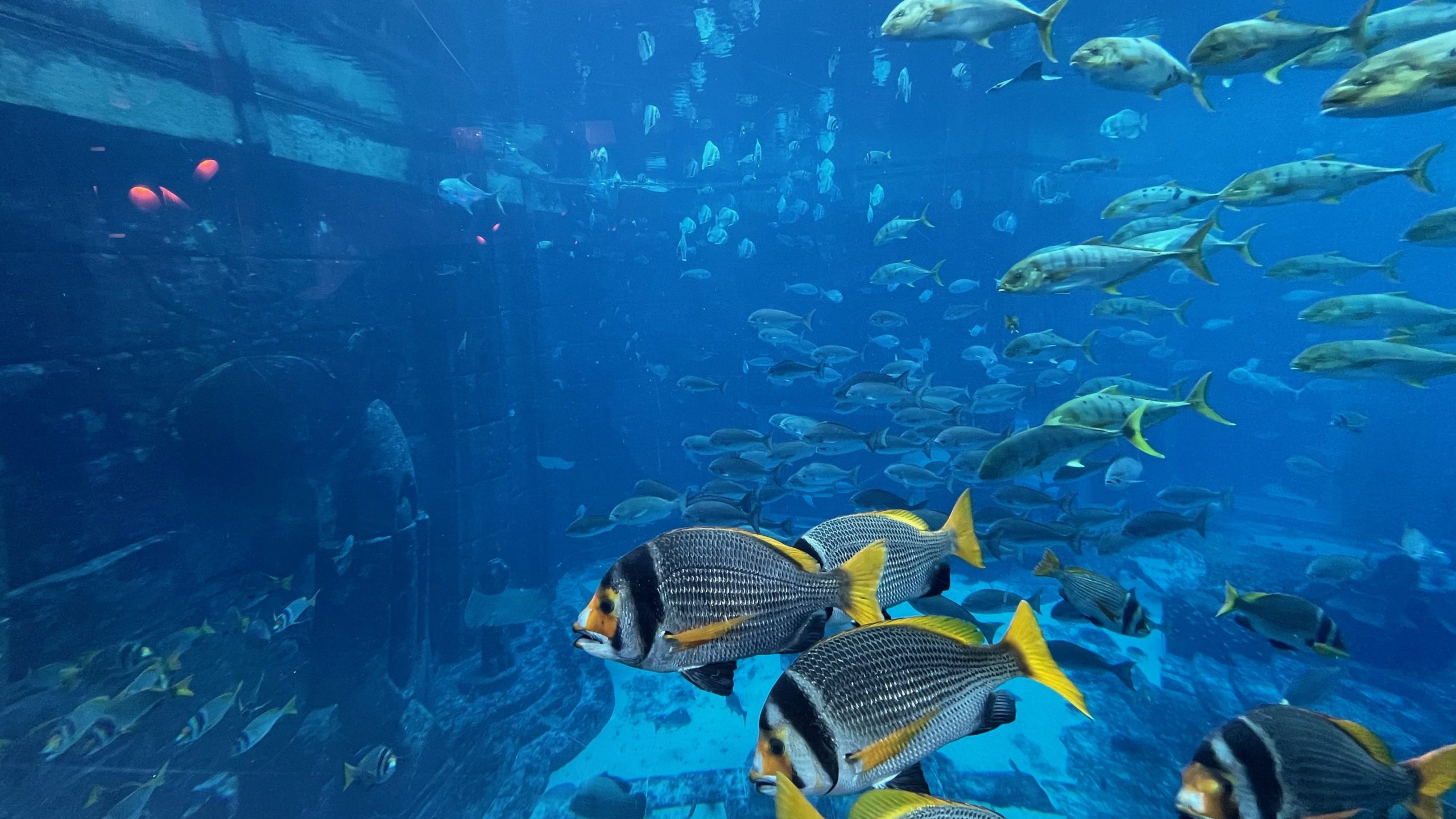This horizontally aligned rectangular photograph captures an underwater ocean scene brimming with aquatic life. In the foreground, there are three to five vividly colored fish, each with silver bodies tinged with light gray, and faces that exhibit a striking blend of yellow with black eyes and a black stripe encircling the top of their heads. Their fins and tails shine a brilliant yellow. The water surrounding them is a vivid, bright blue, lending a refreshing and vibrant feel to the scene.

On the left side of the image, a slightly blurred structure resembling a building made of horizontal rectangles, possibly bricks, is visible. This structure has black or dark-colored portions and appears to have windows on top. Swimming towards this structure are numerous fish, creating a sense of motion and life.

In the background, the water is teeming with countless other fish, most appearing gray or faded light blue, giving depth to the photograph. Additionally, some of the fish to the lower left have black and white bodies with yellow fins. Overall, the photo encapsulates a bustling underwater ecosystem with dynamic colors and varied marine life.